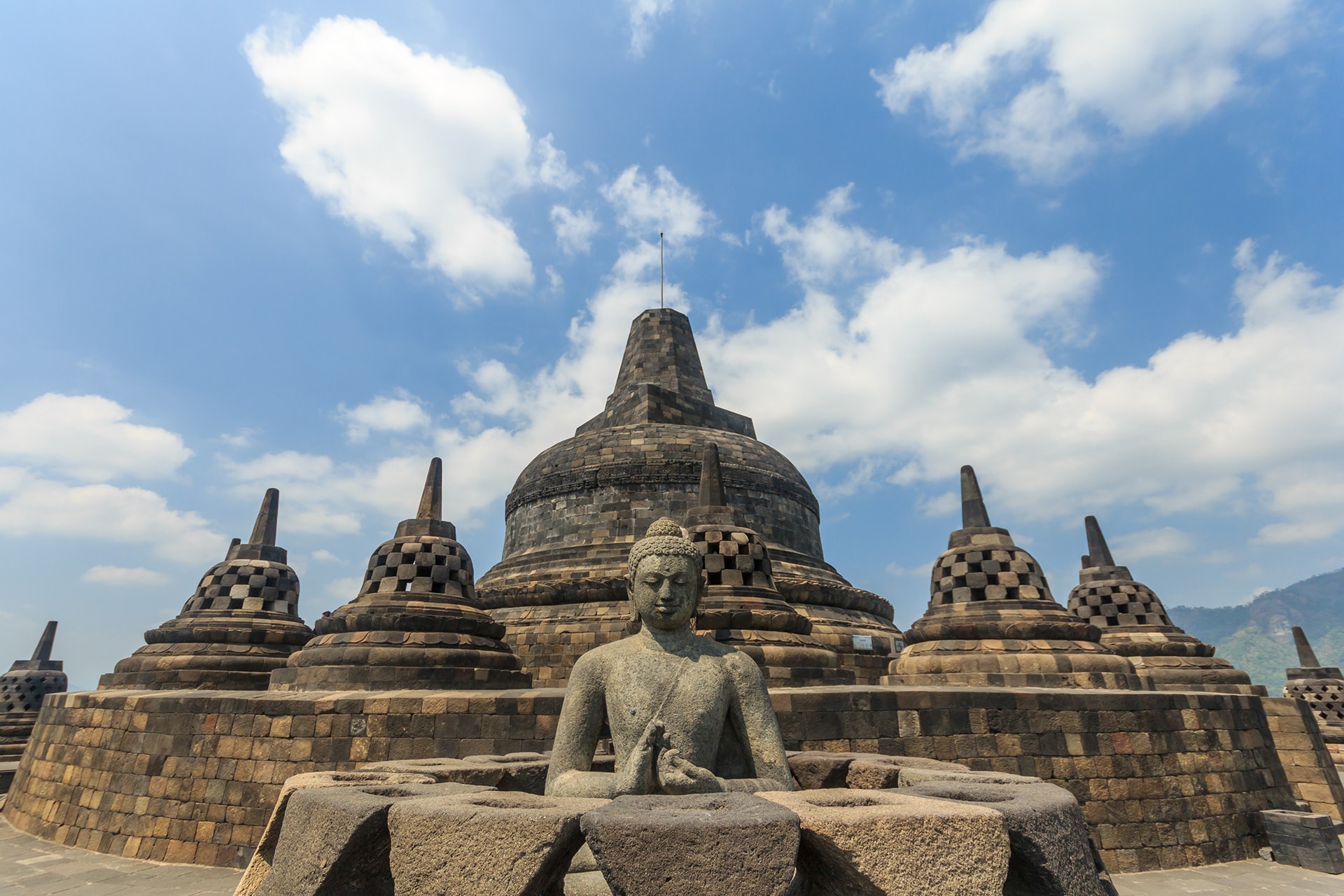This striking photograph captures a serene temple landscape under a radiant, clear blue sky adorned with wispy clouds. The primary focal point is a series of six stone temple structures, each featuring a towering, slightly pointed design that tapers elegantly upwards, reminiscent of the shape of a squeeze bottle. The largest of these structures stands prominently behind the others, its rounded, towering form commanding attention. 

In the foreground, a serene Buddha statue is seated peacefully within a circular arrangement of stone blocks. The Buddha, depicted with closed eyes and a calm expression, has his hands resting gently at his stomach, adding a sense of tranquility to the scene. The temples themselves have base structures with small square cutouts, and one can see through these to appreciate their intricate designs. 

The sandy or desert-like ground contrasts beautifully with the stone structures, creating a harmonious blend with the sky above. This image, devoid of any human presence, evokes a sense of timelessness and peaceful solitude amidst the grandeur of the ancient stone temples.